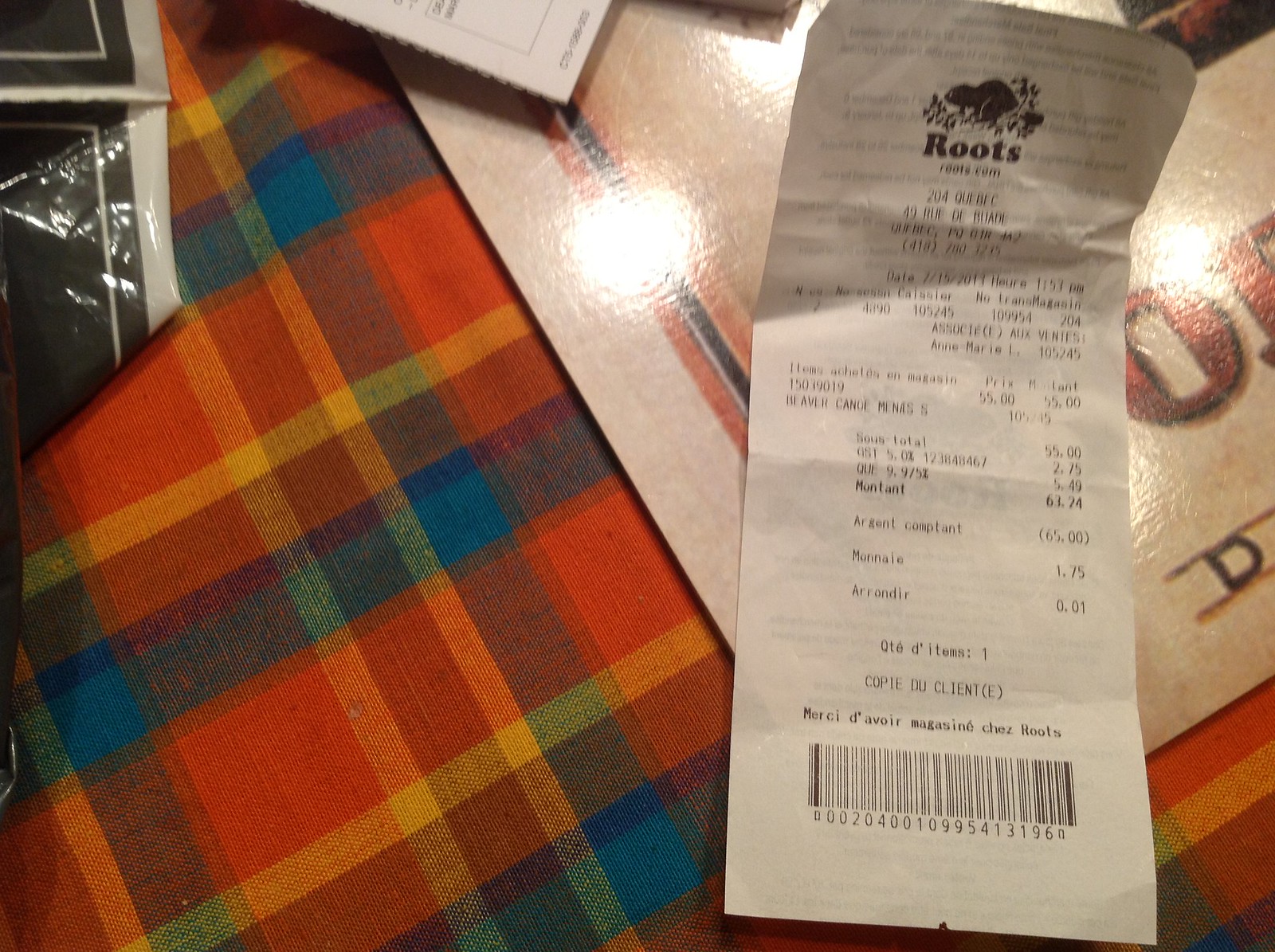The horizontal photograph captures a detailed scene centered around a Roots store receipt dated February 2013 from Quebec. The receipt, which is in French and shows a single purchase of $63.24, is the focal point and lies slightly crinkled and folded on a cardboard object with only the letter "O" visible. This setup rests atop a vibrant plaid tablecloth featuring hues of orange, blue, yellow, purple, red, and brown that evoke fall colors. Surrounding the receipt are various unclear papers and a piece with a red and blue border. In the upper left corner of the image is a small black and white bag, and indoor lighting fills the scene, suggesting the photograph was taken indoors.